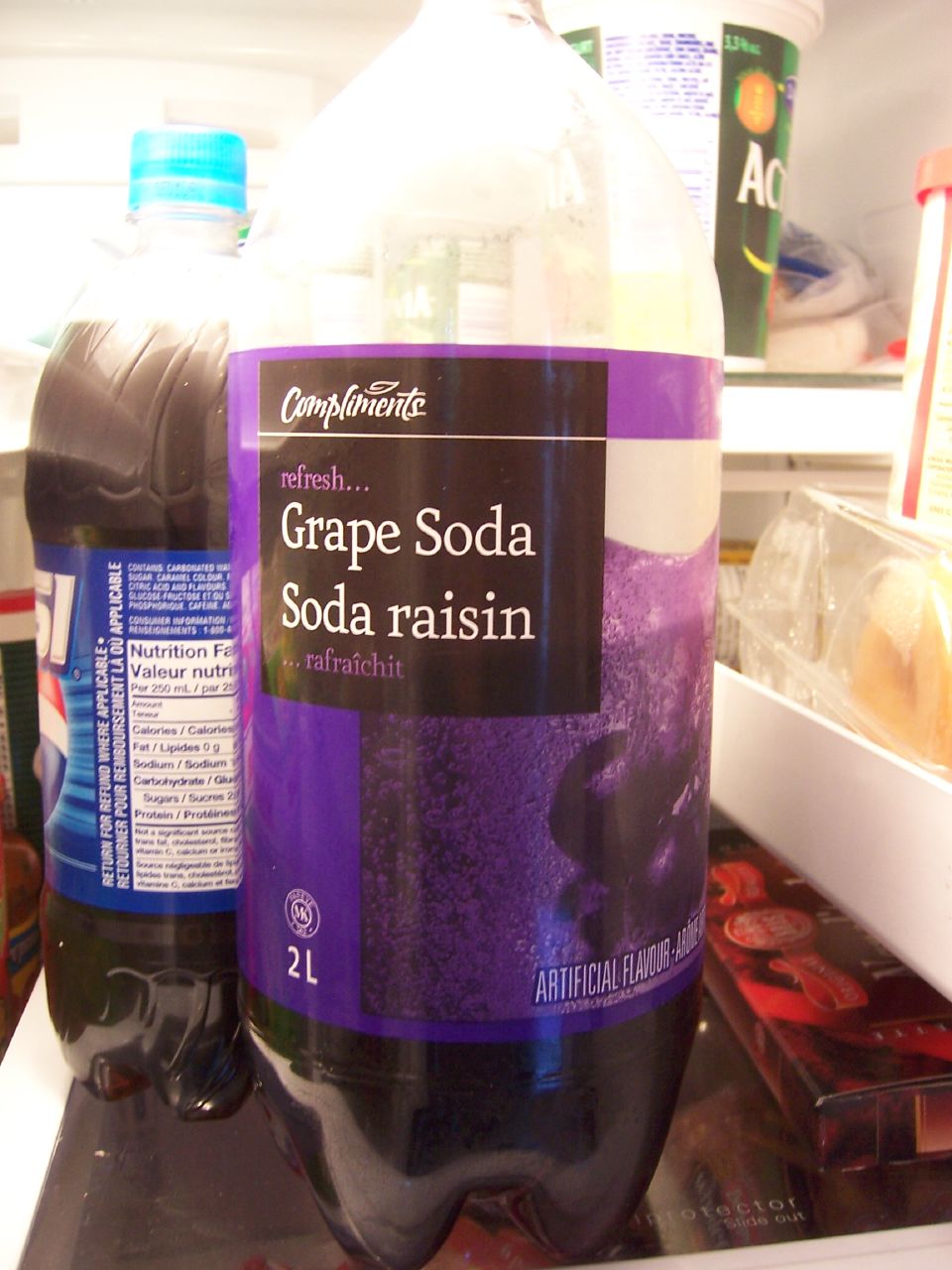A two-liter plastic bottle of grape soda, labeled "Compliments Grape Soda" in white lettering, stands half empty on a kitchen counter. The label, adorned in purple and black hues, also features the words "Soda Raisin," "Refresh," and "Artificial Flavors" at the bottom right. Nearby on the left, an unopened bottle of Pepsi, complete with its blue cap and visible nutritional label, adds contrast to the scene. The setting, either a kitchen counter or potentially a refrigerator, provides a backdrop for these beverages, reflecting a moment of everyday life.